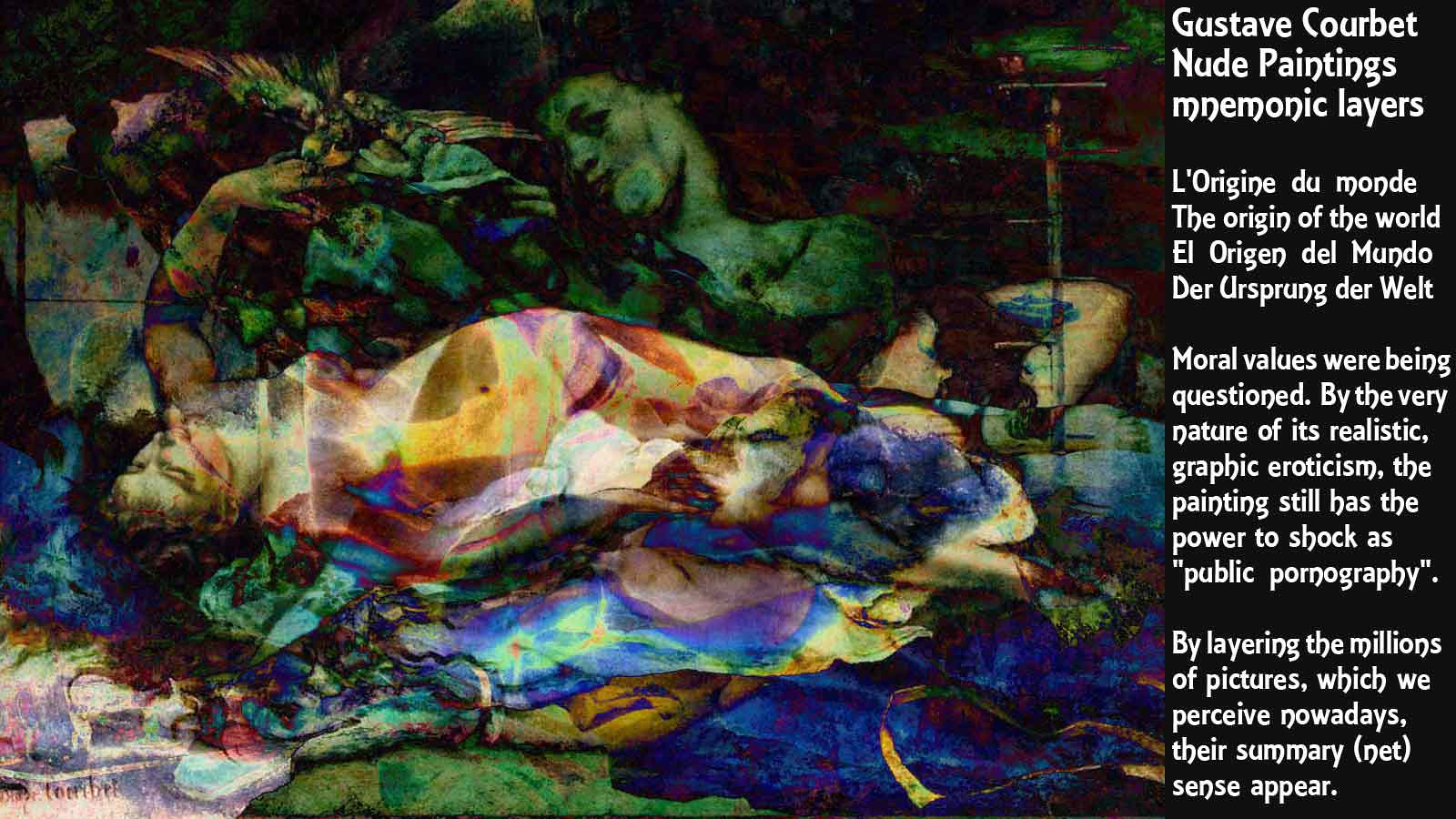The image is an informational slide featuring a painting by Gustave Courbet, prominently showcasing a nude woman lying down with her left arm slightly raised. The artwork is abstract, made up of multiple colors and shapes— including blues, reds, greens, and yellows— creating a complex visual texture with wispy stripes and layers. On the right side, a rectangular section with a black background and white font reads: "Gustave Courbet, Nude Paintings, Mnemonic Layers. L'Origine du Monde, The Origin of the World, El Origin del Mundo, Der Ursprung der Welt." The text also discusses how moral values were questioned by the realistic graphic eroticism of the painting, which still has the power to shock as public pornography. The image captures the essence of the layered and colorful depiction, emphasizing its provocative nature and the ongoing impact of its erotic and realistic portrayal.